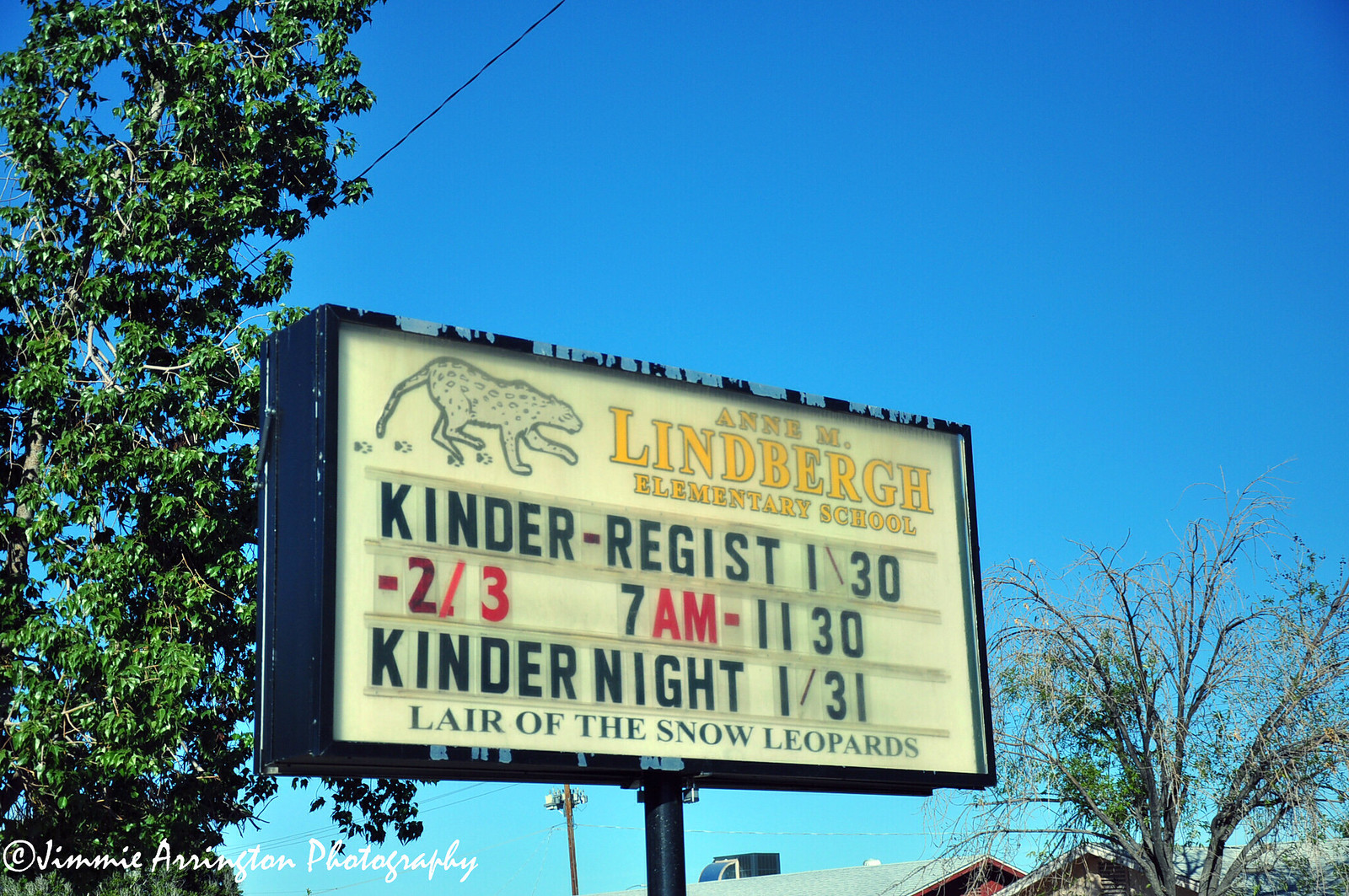In the picture, we see a clear blue sky as the backdrop to a city scene featuring several trees. The trees to the left have green leaves, while the one in the bottom right is mostly bare. A black billboard stands prominently, with text in black, red, and yellow. At the top left of the sign, set against a white background, is an image of a leopard walking with paw prints trailing behind it. The billboard reads "Anne M. Lindenburg Elementary School" in yellow. Below, in black text, it announces "Kinder Register 1-30 to 2-3, 7am to 11:30," and in red, "Kinder Night 1-31." The sign also bears the phrase "Lair of the Snow Leopards." A telephone line stretches across the clear sky, and the photo is credited to Jimmy Arrington Photography in white text on the bottom left corner.